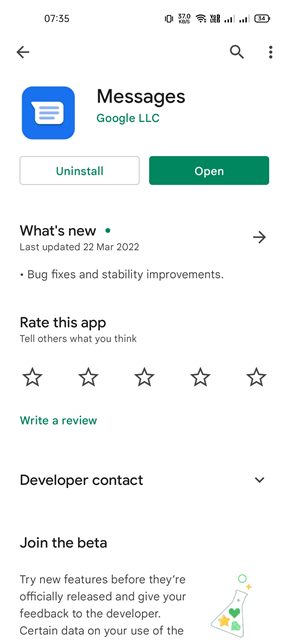This is a screenshot of a smartphone screen displaying the Google Messages app on a white background. In the top left corner, the time is shown as 7:35 AM/PM. The top right corner features status icons, including Wi-Fi, network signal bars, and battery level.

Below the status bar, on the left side, there is a back arrow, and on the right side, there are a search tool (magnifying glass icon) and a vertical three-dot menu icon.

The main section of the screen shows the Google Messages app details. On the left side is the app icon, a blue box with a white piece of paper inside it. Next to the icon, the app name "Messages" is displayed, followed by "Google LLC" in green.

Two pill-shaped buttons provide the options to manage the app: "Uninstall" on the left and "Open" on the right. The "Open" button is selected, highlighted in green with white text.

Below these options, detailed information about the app is listed in four categories:

1. "What’s New": Last updated on 22 March 2022, with notes about bug fixes and stability improvements.
2. "Rate this app": Encourages users to rate the app, featuring five black stars that can be filled in and an option to write a review.
3. "Developer Contact": Has a dropdown menu for additional contact information.
4. "Join the Beta": Offers a description about trying new features before they are officially released and providing feedback to the developer. This section is partially cut off but includes an illustration of a scientific beaker with three icons inside it—a yellow star, a green heart, and a geometric figure.

The overall arrangement and detailed icons provide a clear and user-friendly interface for managing the app on the phone.